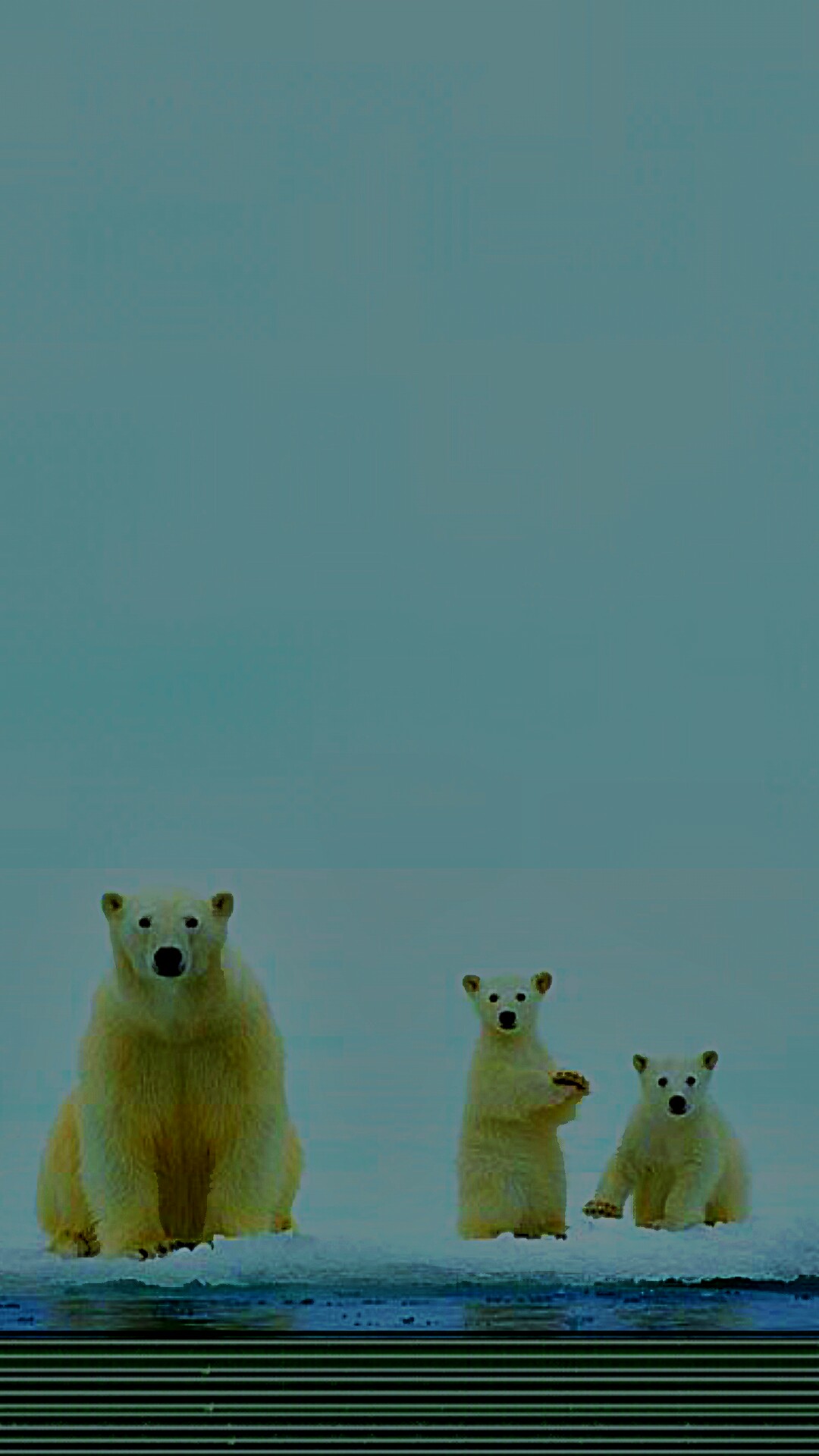This is a horizontally oriented photograph of a mama polar bear and her two cubs, capturing their stark presence against an expansive blue sky. The polar bears are situated towards the bottom of the frame on what appears to be a snowy and icy shore, with hints of wet ground and possibly a grated or concrete area where the snow stops. Mama bear, the largest of the trio, is positioned on the left and appears to be sitting, providing a full view of her round, fluffy form. Her fur, like that of her cubs, is a yellow-white rather than pure white, adding a warm tint to their otherwise icy surroundings. The two cubs on the right, smaller and playful yet momentarily paused, are also facing the camera directly. All three bears have black noses, black eyes, and small ears, giving them an irresistibly cute and fluffy appearance as they curiously stare at the photographer. The seamless blend of the blue sky and the snowy background highlights the stark contrast and beauty of the polar bears in their natural habitat.